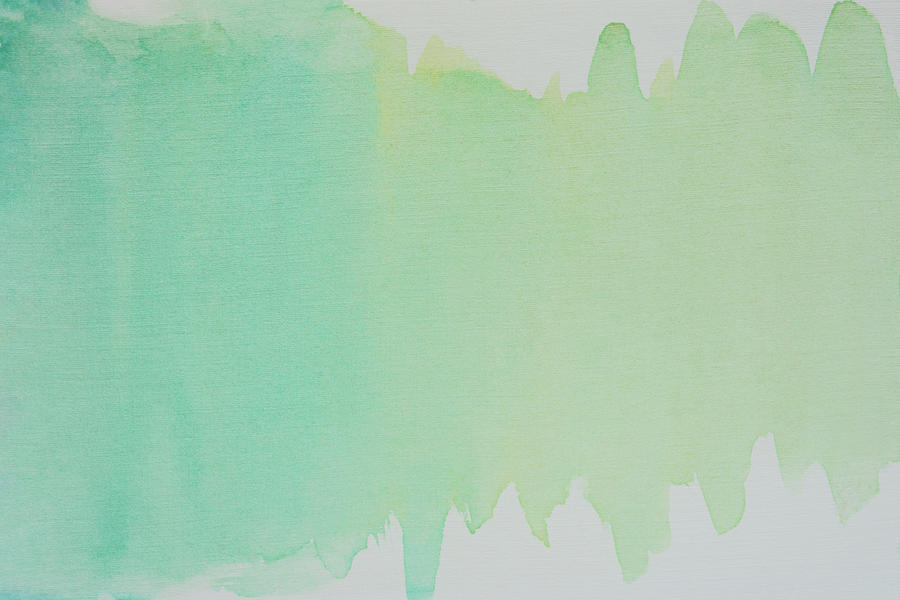This image showcases a horizontal watercolor painting on a gray or light gray background. The painting features vertical streaks in a gradient of colors blending seamlessly from left to right. On the left side, the streaks start with shades of turquoise blue and blue-green, created by wide brush strokes that run from top to bottom. These streaks merge into a central area where blue and green hues intermingle, forming a blended middle section difficult to distinguish as either distinctly blue or green. Moving further right, the colors transition into lighter shades of lime green and green-gold. Throughout the right side, there are additional brush strokes that expose more of the paper beneath, giving it a faded, textured appearance. The overall composition is abstract, with no specific pattern, characterized by the artist's repetitive vertical brush movements.